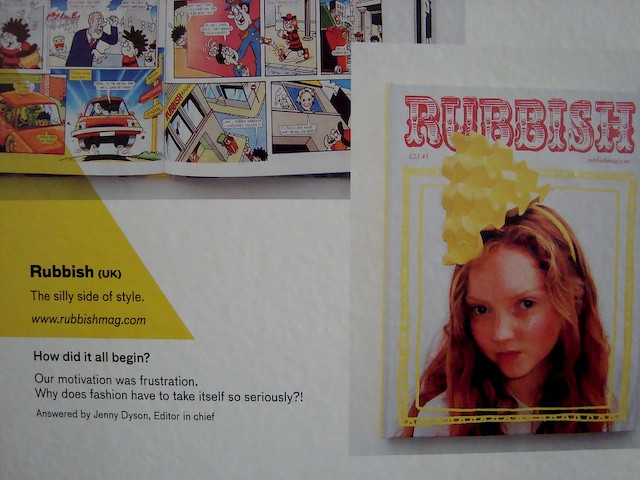The image displays a visually compelling advertisement for "Rubbish" magazine, positioned against a plain white background. Dominating the right side, there's the cover of the magazine featuring a red-haired girl adorned with a yellow headband that has a geometric flower design. Above her, the bold red title "Rubbish" stands out. To the top left, there’s an open comic book, specifically the British version of Dennis the Menace, adding a playful touch. On the left, striking text reads, "Rubbish UK, the silly side of style," along with the website "www.rubbishmag.com." The text also includes a reflective quote from Editor-in-Chief Jenny Dyson: "How did it all begin? Our motivation was frustration. Why does fashion have to take itself so seriously?" This advertisement blends whimsical visual elements with insightful commentary, encapsulating the magazine’s unique and irreverent approach to fashion.